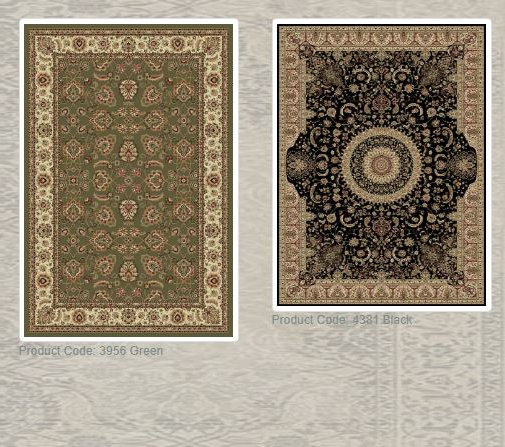The image features a muted rug laid down as the background, with its pattern subtly visible but not dominant. Two additional rugs are placed on top of this background. The rug on the left showcases a harmonious blend of green, cream, red, and various shades of brown. It is bordered with a distinct white edge that appears digitally created. To the right, the second rug displays a rich palette including black, multiple browns, a rusty red, and hints of orangey brown, also edged with a similar white border.

Beneath the left rug is the text "product code 3956 green" in a light gray font that blends slightly with the muted background. Similarly, beneath the right rug is the text "product code 4381 black," also in light gray. The rug on the left is vertically oriented and appears longer, while the rug on the right is horizontally oriented, slightly wider, and gives an impression of being just a tad bit larger, though this could be an optical illusion. There is no additional context or indication of the source or website associated with these items.